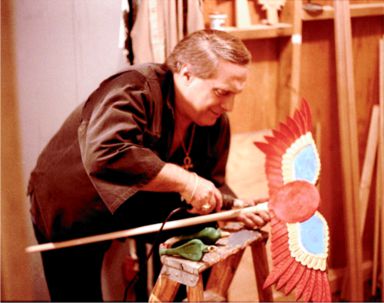This vintage photograph, likely dating from the 70s or 80s, depicts a middle-aged man with short brown hair and a brown shirt that reaches halfway down his forearms. He is working on a colorful project that appears to be a lawn ornament, specifically a butterfly, with vibrant red, blue, yellow, and white feathers or wings. The butterfly, which features a distinctive lollipop-like center, is attached to a long wooden pole he holds horizontally. The man, wearing a bracelet on his arm, is leaning against a wooden stepladder, meticulously using a plugged-in tool, possibly a glue gun. In the background, the image shows an unfinished interior space with wooden walls bearing some shelves, loose two-by-fours, and various unidentifiable green objects scattered on a nearby workbench. The overall brownish tint of the photograph, along with the man's attire and the ambience, evokes a nostalgic feel typical of the era.